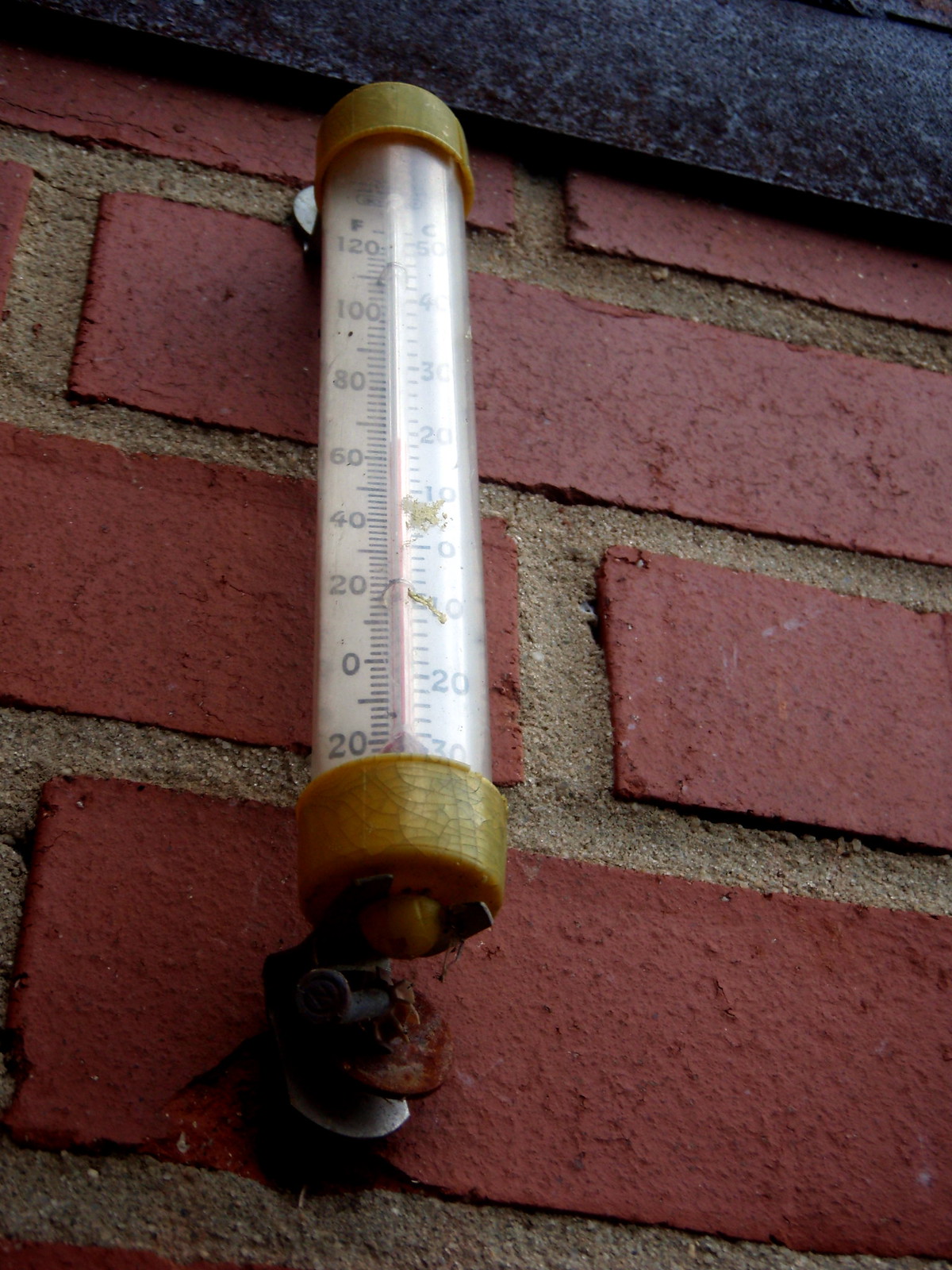The photo captures a close-up view of an old-school mercury thermometer mounted on a red brick wall. The thermometer is secured to the wall with two metal hinges, bolted at the top and bottom into the thick, gray concrete grout lines that separate the bricks. The bricks are an earthy red tone, and the thick grout lines emphasize the rustic texture of the wall. Positioned above the photographer's eye level, the thermometer is encased in a sleek glass cylinder with elegant gold caps at the top and bottom. The thermometer features a traditional vertical display, with Fahrenheit measurements on the left and Celsius (Centigrade) on the right. At the top of the image, a black stone header or molding adds a touch of architectural detail, framing the scene.